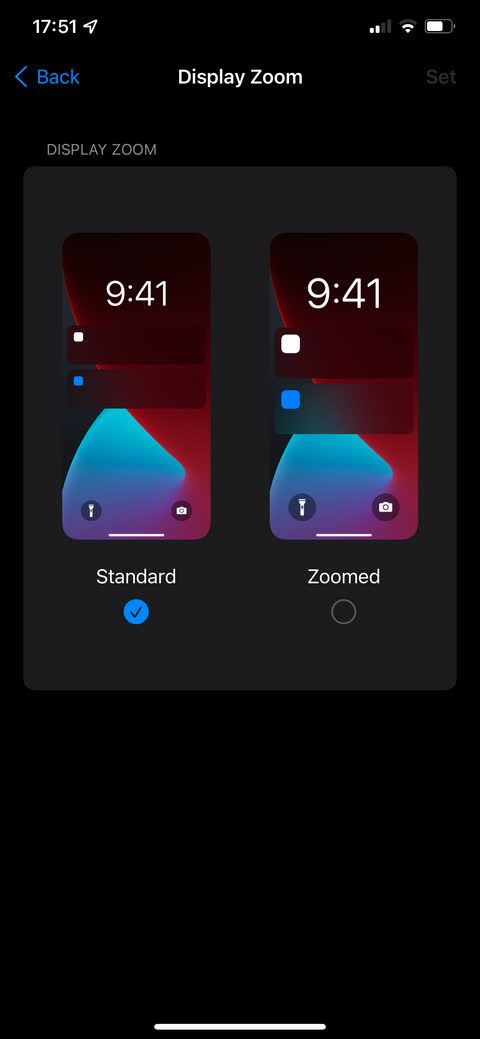This portrait-oriented screenshot, taken from a phone, features a plain black background. At the top, the white text "1751" denotes the time, accompanied by a small rightward-pointing arrow. The top-right corner displays icons for WiFi signal, battery, and data signal.

Central to the screenshot is the "Display Zoom" settings page for the phone. The title "Display Zoom" appears at the top in white text. To its left, the word "Back" in blue, preceded by a leftward-pointing blue arrow.

Below the title, a grey box distinguishes itself from the rest of the page. Inside this box, two side-by-side images demonstrate different versions of the phone's display: "Standard" and "Zoomed". Below the images, a blue circle check mark indicates that the "Standard" option is currently selected. The grey text "Display Zoom" labels the top of this box.

Both phone images within the grey box display the time "941" in white text, set against a red and blue patterned background. They each show two example notifications: the left being smaller and the right larger, highlighting the difference between the "Standard" and "Zoomed" views.